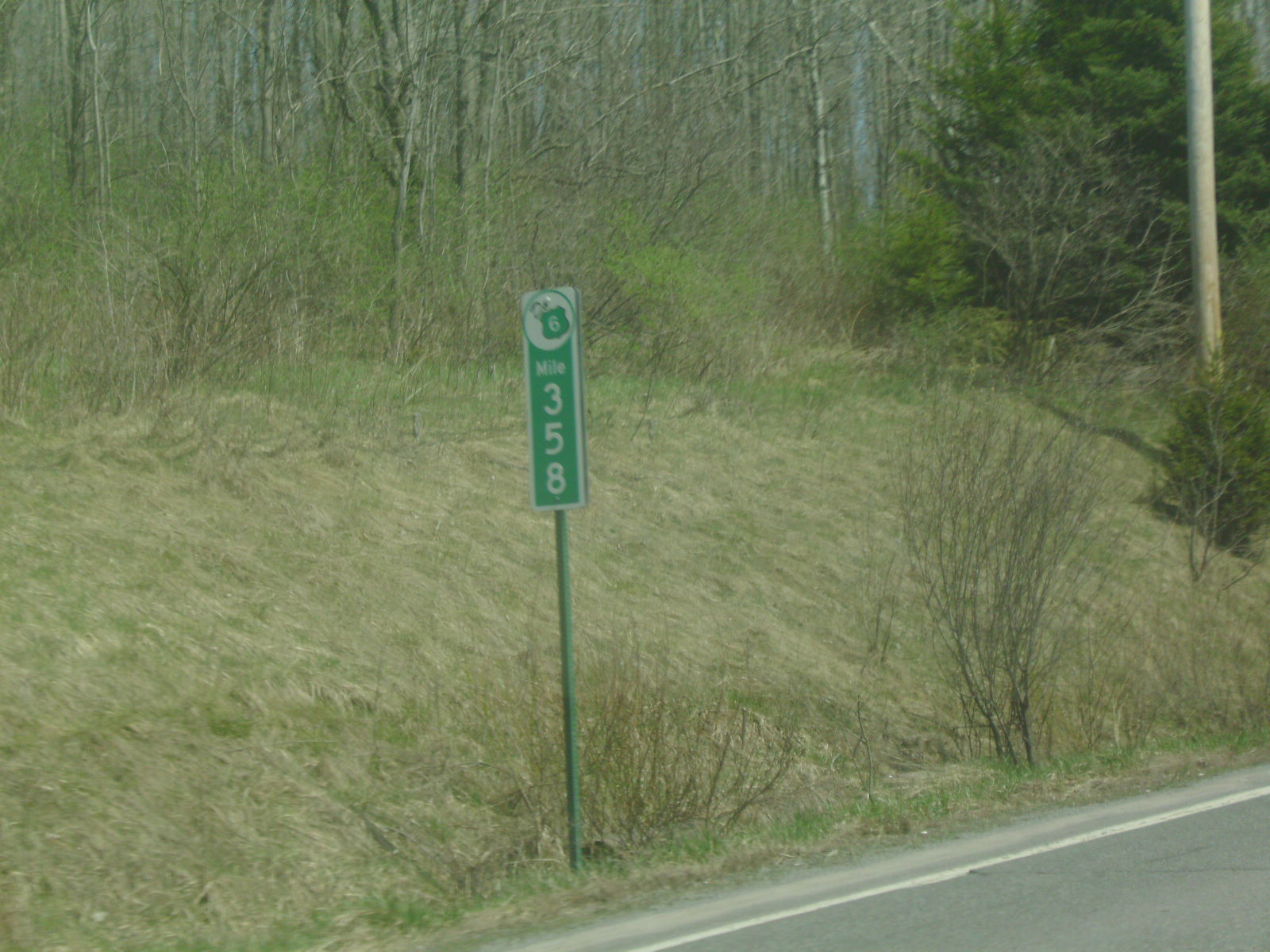This image depicts a scene captured from inside a car, looking out the window to the left. It showcases a stretch of a highway bordered by a grassy embankment and a dense forest. The asphalt road is partially visible at the bottom-right corner, featuring a white stripe marking the edge of the shoulder. Prominently positioned near the roadside is a green pole with a vertically rectangular sign. The sign has a white outline and reads "Mile 358" in white letters against a green background. Above this, there's a small white circle containing the number 6. The surrounding landscape gives off an autumnal or wintry atmosphere, with thin, leafless tree trunks and an abundance of dry, sparse brush and bushes. The area at the base of the pole is particularly brushy, adding to the overall rustic feel of the scene.